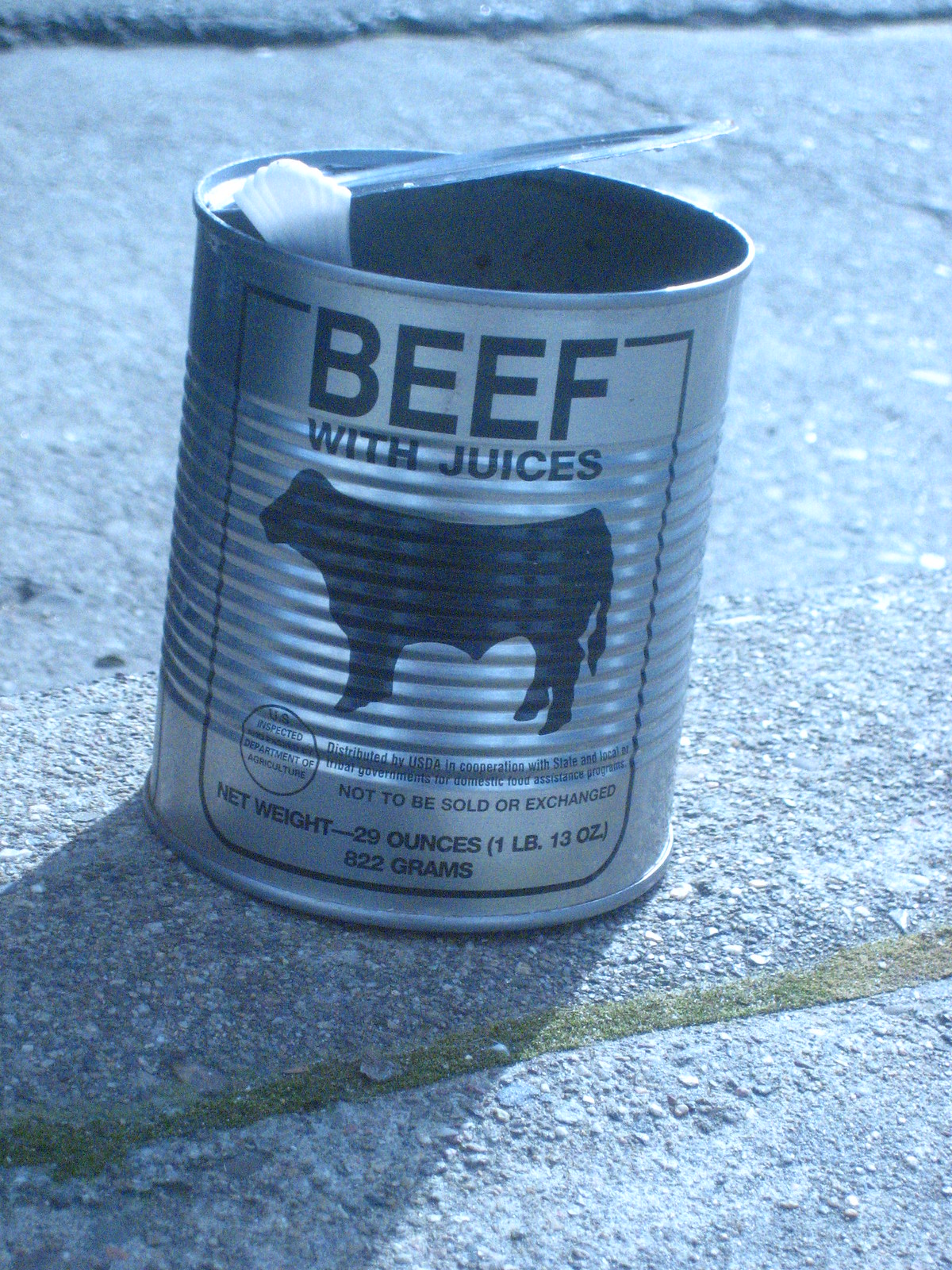The image depicts an open silver can of beef with juices sitting outside on a gray sidewalk, evidenced by the shadow and a yellow worn stripe in front of it. The can's lid is tilted upwards, revealing its contents. A black illustration of a cow facing left is prominently displayed on the label, which features a black border around the cow. The text on the label includes "beef with juices" and a sentence prohibiting the sale or exchange of the item. Further text details the net weight as 29 ounces (1 pound and 13 ounces or 822 grams). Additional labeling indicates it is distributed by the USDA in cooperation with state and local tribal governments for domestic food assistance programs, with the U.S. Department of Agriculture's inspection mark on the lower left of the can.